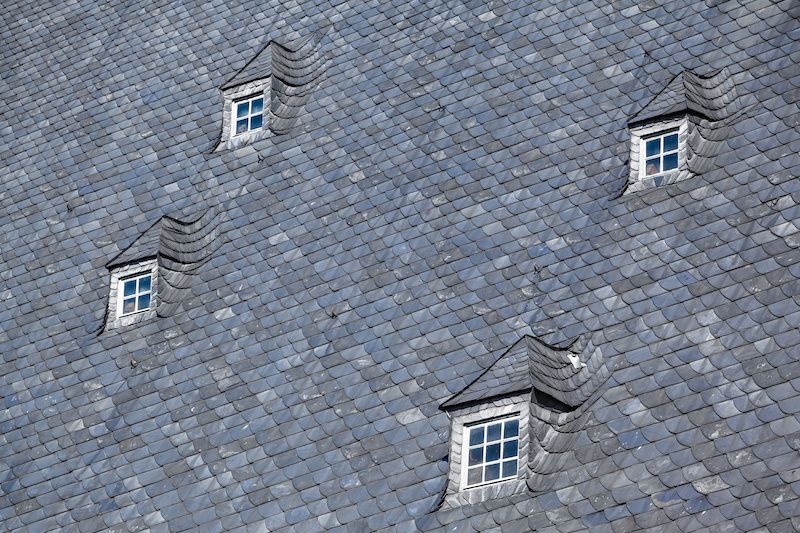This digitally manipulated photograph features a large, gray shingle roof, reminiscent of fish scales in texture and stone-colored in appearance. The roof is adorned with four dormer-style windows, each emerging prominently. These windows, appearing unevenly spaced with varied elevations, are a focal point of the image. The most distinctive window, located bottom center-right, is larger with nine panes of glass and appears distorted as it slants and melts unrealistically into the roof. The other three windows, each fitted with four panes of glass, are strategically repeated throughout the composition, suggesting heavy clone stamp editing. This repetition includes placements closer to the top right corner, left center, and slightly lower on the left side of the roof. The image itself is wider than it is tall, offering an intriguing yet surreal depiction of a roof that combines elements of architectural realism with noticeable digital alterations.